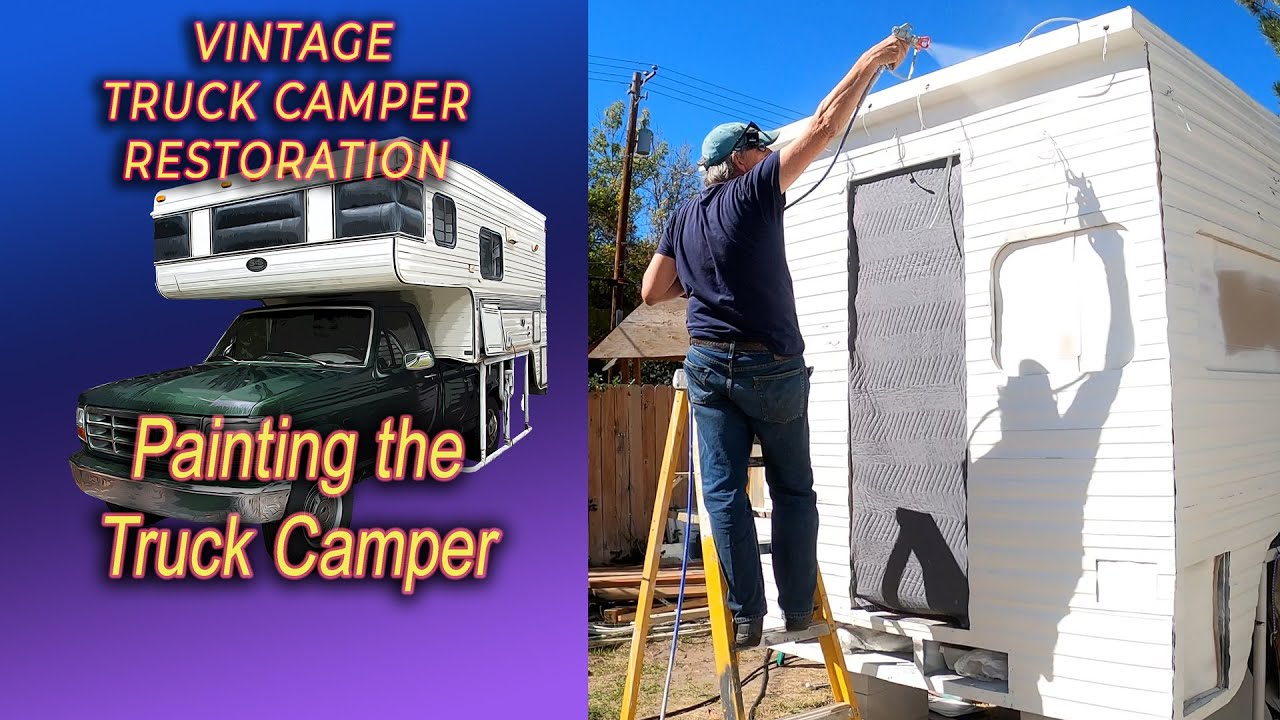The image is a flyer for "Vintage Truck Camper Restoration," prominently displayed in yellow text on a purple background in the upper left corner. Below this heading, it states "Painting the Truck Camper." The focal point is a green truck with a camper integrated into its bed, extending above the cab. To the right of the truck, the image seamlessly transitions to a photograph of a man on a yellow and gray stepladder, spraying water or paint onto a white camper. The man is clad in blue jeans, a brown leather belt, a short-sleeved purplish-blue t-shirt, and a ball cap. He appears to be engaged in restoring or cleaning the camper, suggested by the action of spraying water. The camper features a gray door on the back, and the scene is set against a backdrop of a wooden fence, a clear blue sky, and visible power lines.